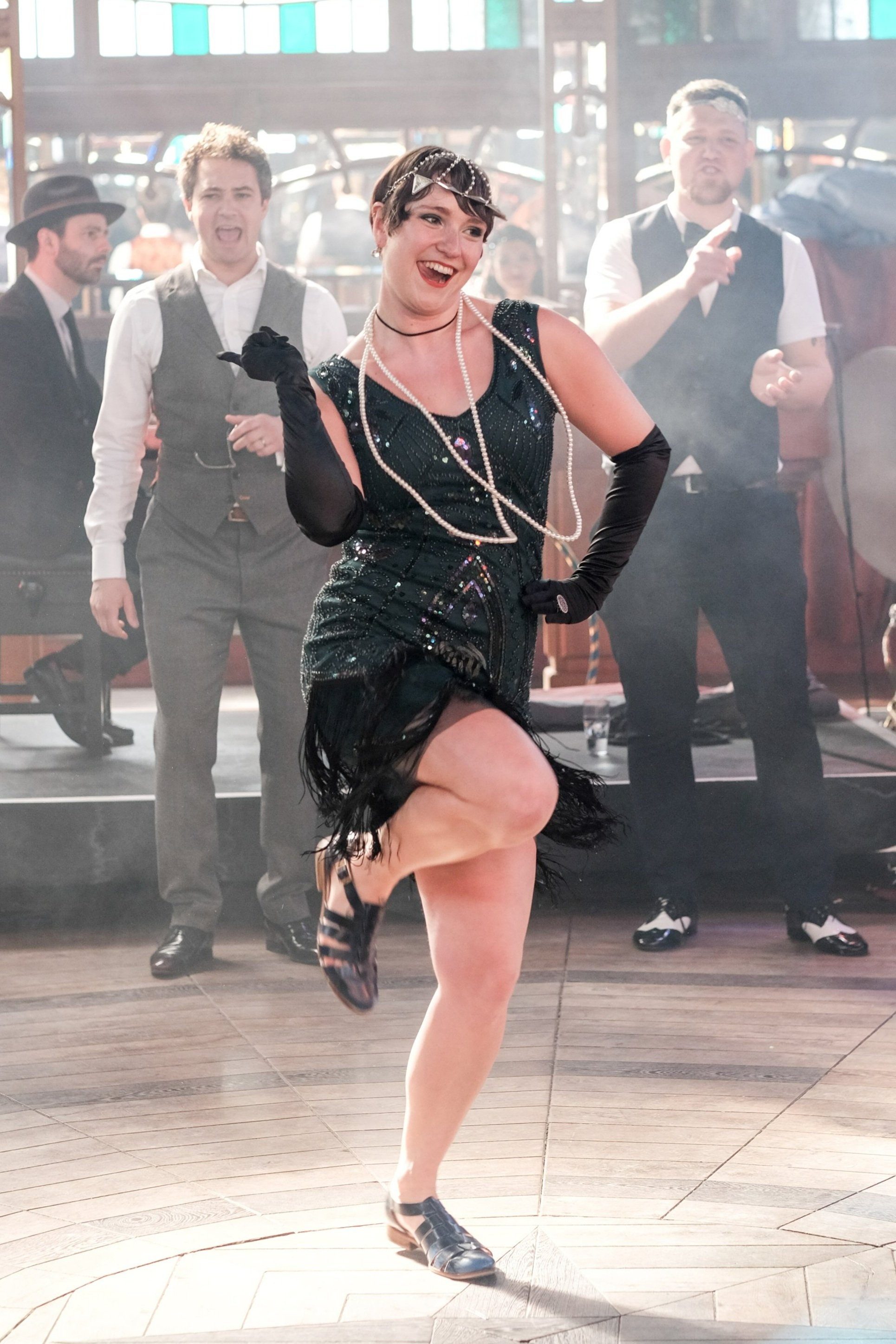The image captures a lively scene centered around a woman dressed in an authentic 1920s flapper style. She wears a black sequined dress that falls to her thighs and pairs it with long black gloves extending to her elbows. Her outfit is accessorized with two long pearl necklaces that reach down to her stomach, strappy black shoes, and an elaborate headpiece adorned with strands of pearls cascading down. She is energetically dancing on a wooden floor, her left leg grounded while her right leg is raised in the air. Her left arm rests on her hip, and her right arm is lifted in a lively motion. She faces forward but looks off to the right, showcasing an open-mouth smile with visible top teeth. 

In the background, three men are sharply dressed—two in suits without coats appear to be part of the scene, possibly watching or participating. A third man, seated further back, wears a full dark suit and hat, seemingly involved with a piano or similar instrument. This setting appears to be a modern reenactment of a 1920s scene, likely taking place during the day on a performance floor, with a building visible behind them.